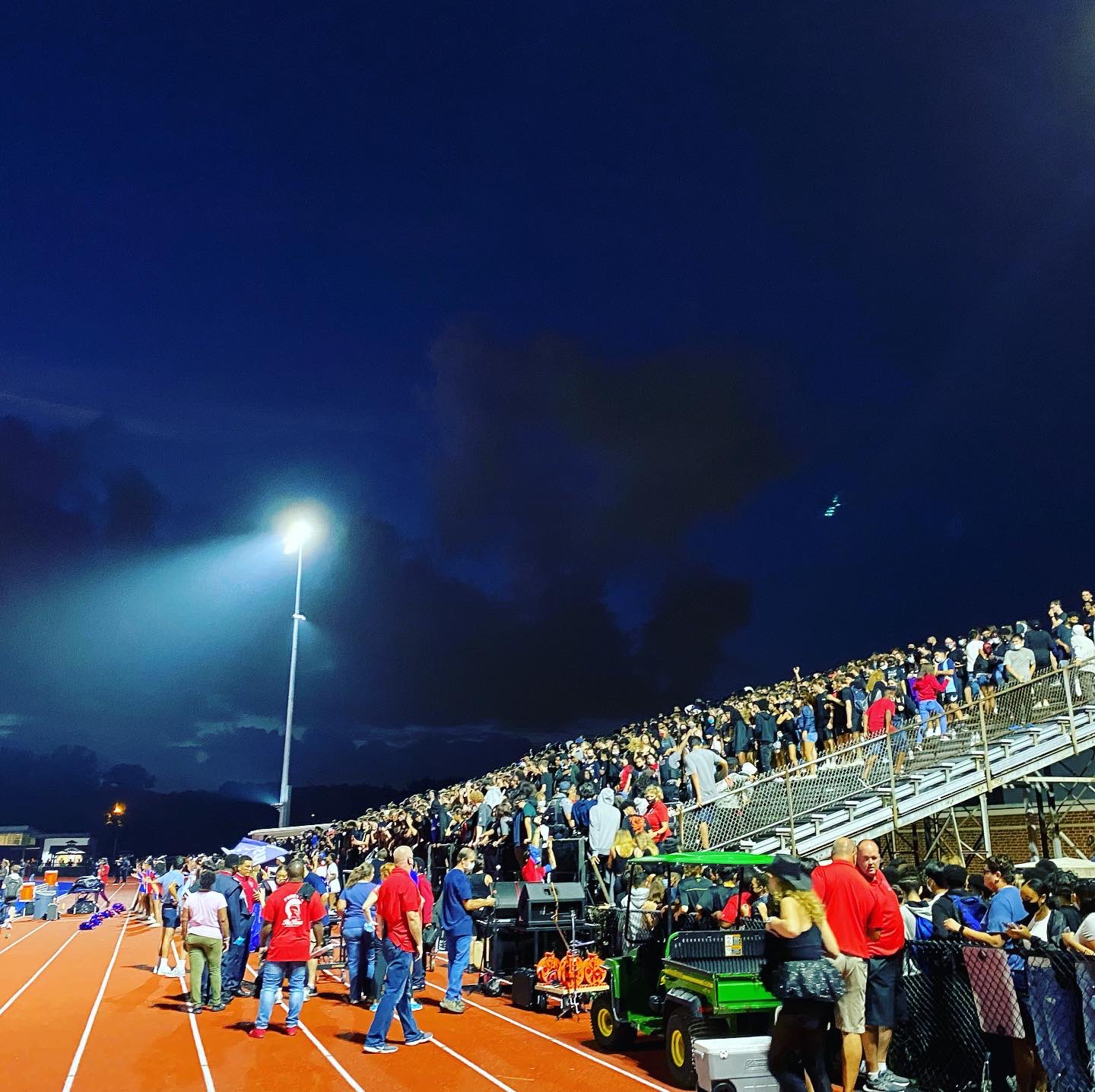This high-quality nighttime image captures the vibrant atmosphere of a high school football game. The stands, located on the right-hand side, are filled with around 400-500 enthusiastic fans, and more people are seen filtering in. The bleachers rise gradually about 40 to 50 feet into the night sky, which is a deep dark blue with large puffy clouds. A tall light pole stands at the center back of the stadium, casting bright light over the crowd and the field. In front of the stands is a track and field area where people are mingling, barbecuing, and enjoying soft drinks. There's a row of barbecue grills chained together on the track, along with a green John Deere tractor that seems to have delivered coolers for the event. Additionally, the scene shows the backside of a bench with coolers, chairs, and pom-poms scattered on the ground, indicating a lively cheerleading presence. The dark blue sky in the background contrasts against the well-lit stadium, with distant hills and trees adding to the picturesque setting.